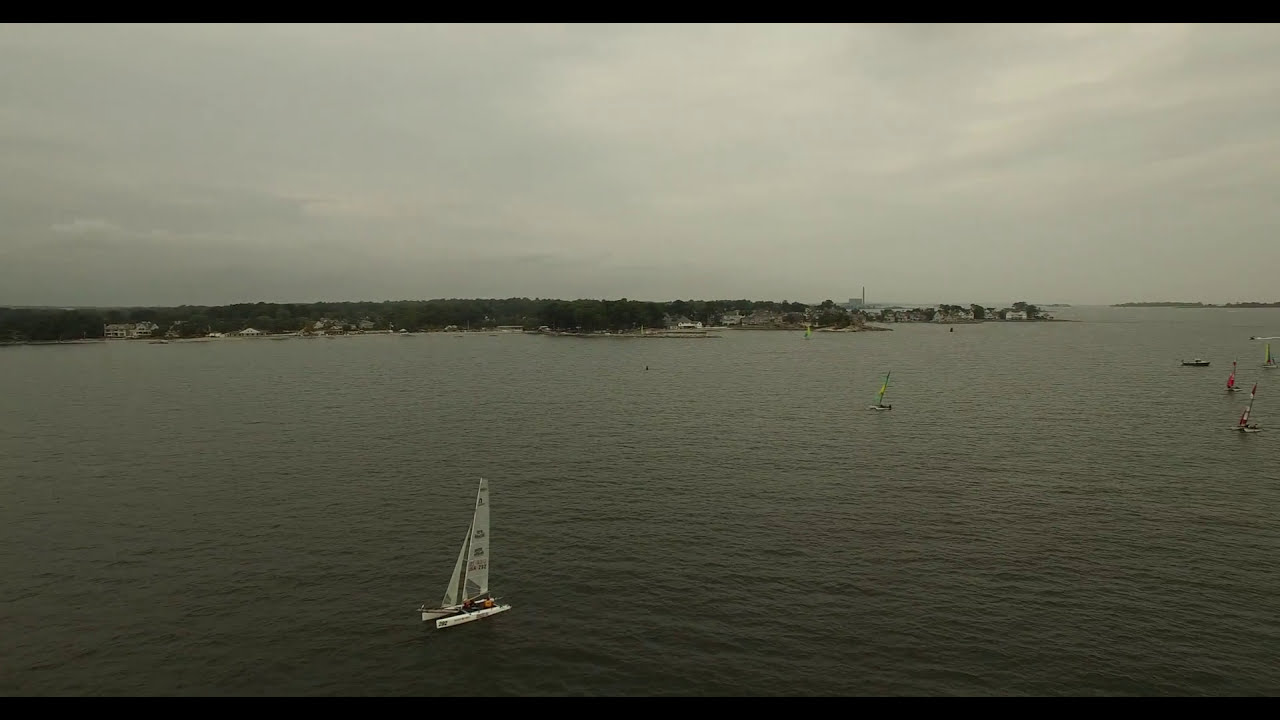This vivid photograph captures a serene scene on a large body of water under an overcast sky. The water, appearing black and gray, mirrors the cloudy atmosphere of either early morning or late afternoon. Dominating the center-left is a sleek catamaran, identifiable by its white pontoons and dual sails. Scattered across the water are several other sailboats, including ones with bright green, yellow, and red sails, suggesting a possible regatta. In the backdrop, a slender strip of tree-covered land stretches from the left to the center, revealing patches of tall, bushy green trees and modest buildings, perhaps small neighborhoods or office parks. The right side of the photo shows more low-lying land with additional trees and piers, enhancing the tranquil yet mysterious feel of the scene.